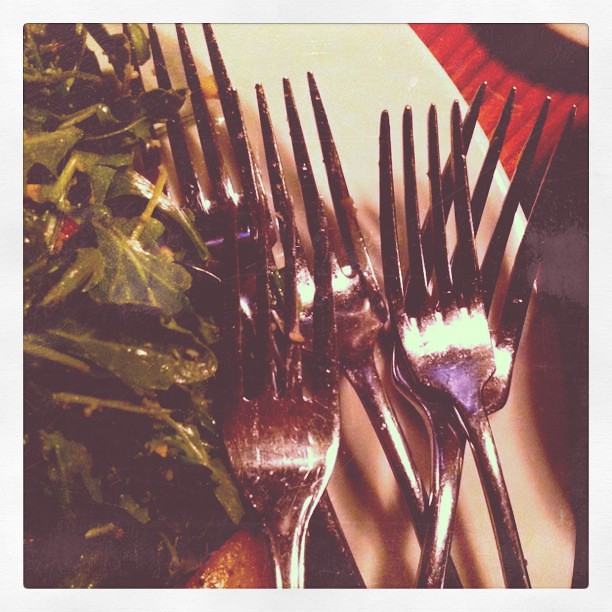The photograph showcases a vibrant food table scene, centered around five silver, four-pronged metal forks that are neatly stacked on a white plate. The light gray border frames this main image, emphasizing the glistening cutlery. Positioned on the left of the plate is a fresh green salad made up of leafy vegetables, which appear to be moist or dressed, adding a tantalizing shine. The plate itself rests on a tabletop characterized by light red wood with dark brown grain patterns. In the upper left corner of the image, a small portion of another matching plate or dish is visible, indicating the presence of more tableware. The ambient light reflects off the metallic forks, further enhancing the photograph's lively and appetizing atmosphere.